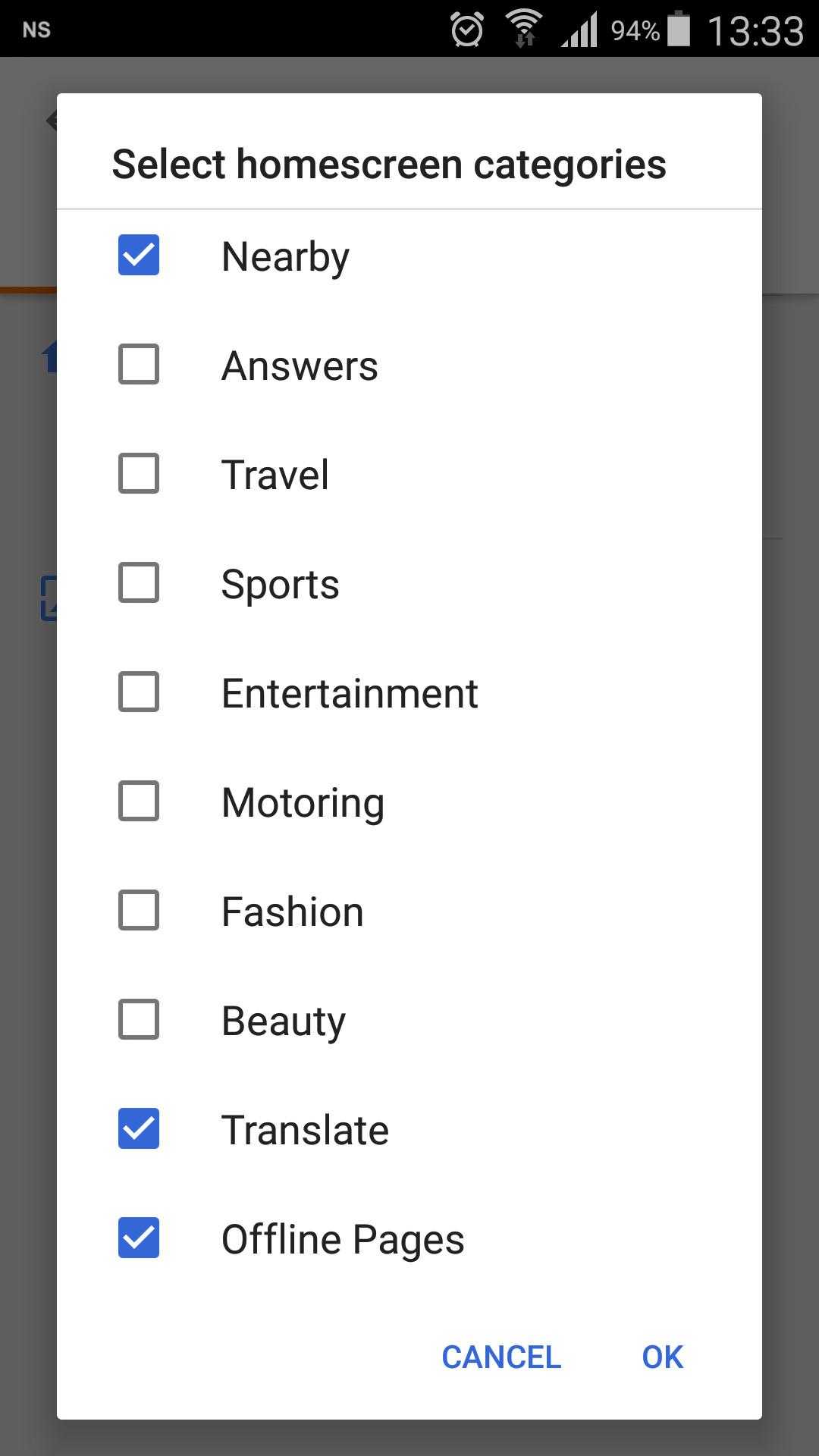A phone screenshot displaying a pop-up window for selecting home screen categories. The pop-up window is white, long, and narrow with the title "Select Home Screen Categories" at the top. Below the title is a checklist featuring ten categories: Nearby, Answers, Travel, Sports, Entertainment, Motoring, Fashion, Beauty, Translate, and Offline Pages. Each category has either a checkbox or an empty square to its left. The categories Nearby, Translate, and Offline Pages are marked with blue checkboxes, indicating they are selected, while the rest remain unchecked. At the bottom of the window are two blue buttons labeled "Cancel" and "OK" towards the right. The rest of the screen appears darkened. In the top right corner of the phone screen, the time reads 13:33, and the battery level is at 94%.